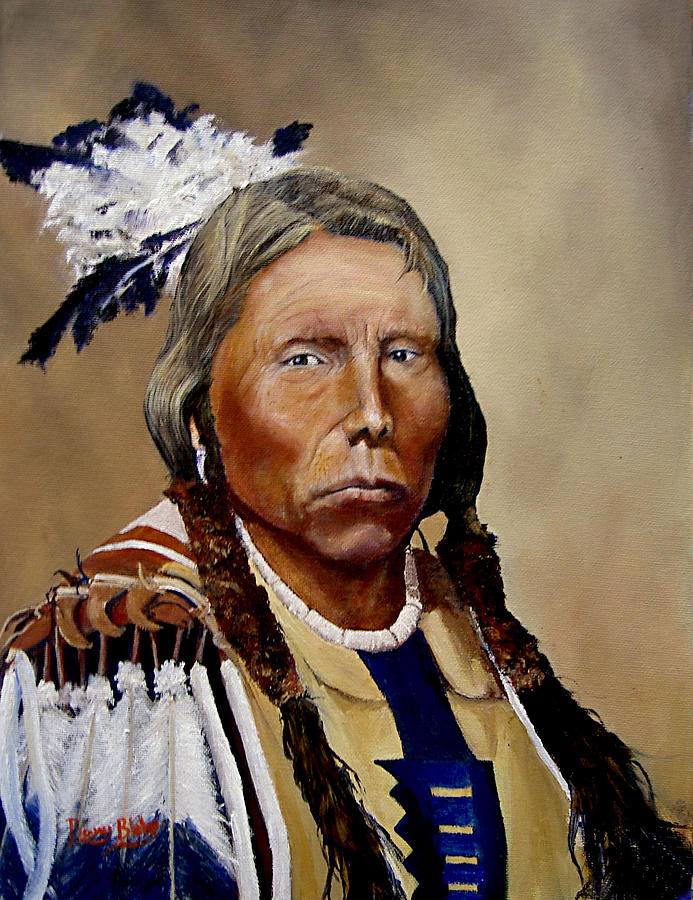The painting depicts an elderly Native American man, most likely in his 60s or 70s, characterized by his stern and weathered expression. His deeply furrowed brows and downturned lips convey a solemn and serious demeanor. He has long braids that drape over his chest, with the ends of the braids covered in black. The man's hair is predominately gray, signifying his age. He wears a traditional regalia that includes a tan garment, likely a hide, adorned with a blue and yellow striped fabric down the front. His clothing is intricately decorated with multiple feathers—both black and white as well as blue and white—as well as animal teeth, which are brown in color. A prominent white shell necklace is visible around his neck. The feather plume is especially notable, positioned at the back of his head and adding to the authenticity of his cultural attire. The man has light brown skin, a narrow and long nose, and dark, profound eyes. The portrait captures him standing and facing the viewer head-on, his expression imbued with a sense of gravitas, reflecting not just his age but his heritage and the weight of his experiences.